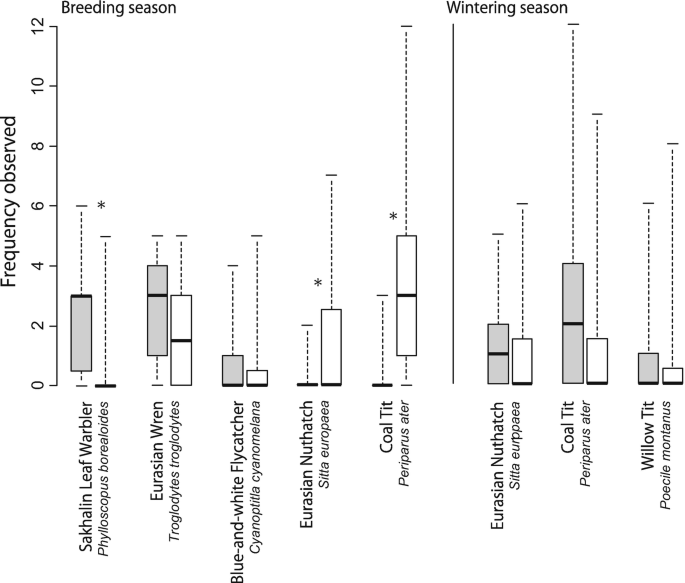The image displays a detailed bar chart on a plain white background, utilizing a landscape orientation and black-and-white color scheme. On the left-hand side, a vertical axis labeled "Frequency Observed" ranges from 0 to 12, marked in increments of two. The top of the chart divides into two sections: "Breeding Season" on the left and "Wintering Season" on the right. 

Below this, the chart features a series of labeled bars corresponding to different bird species. Each species name is written sideways. Starting from the left, under the "Breeding Season" section, are the Sacculine Leaf Warbler (Phylloscopus borealoides), Eurasian Wren (Troglodytes troglodytes), Blue and White Flycatcher (Cyanomelana cyanomelana), Eurasian Nuthatch (Sitta europaea), and Coal Tit (Periparus ater). Moving to the "Wintering Season" section, it lists the Eurasian Nuthatch (Sitta europaea), Coal Tit (Periparus ater), and Willow Tit (Poecile montanus).

Each bird species is represented by gray and white bars indicating different data points, with gray typically signifying one set of data and white another, though the specific frequencies remain unlabeled. A vertical black line separates the breeding season data from the wintering season data.